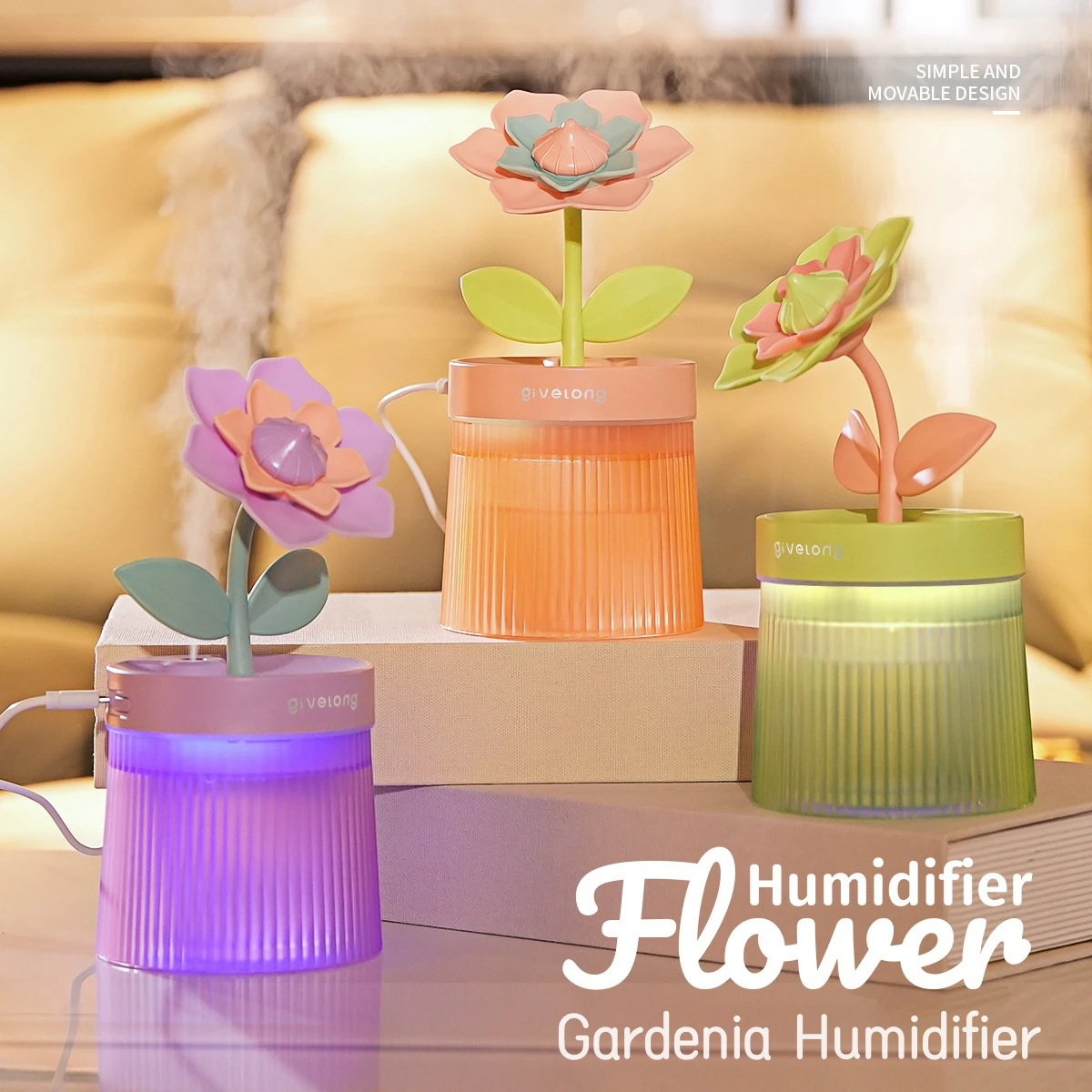This advertisement features three vibrant Humidifier Flowers, specifically the Gardenia Humidifier model, positioned on a coffee table adorned with two books, with a couch visible in the background. Each humidifier mimics a flower growing out of a pot, crafted from semi-opaque plastic. The display includes: a lilac-colored humidifier with matching petals and a peach center, connected by a pale blue stem and leaves; a center orange humidifier with an orange and gray flower atop a green stem; and a green humidifier featuring a peach-colored stem and flower with green elements. All three are emanating steam and two are visibly connected to a power source. The text "Humidifier Flower, Gardenia Humidifier" is displayed prominently in white font in the lower right corner, while the top of the ad boasts "Simple and Moveable Design."